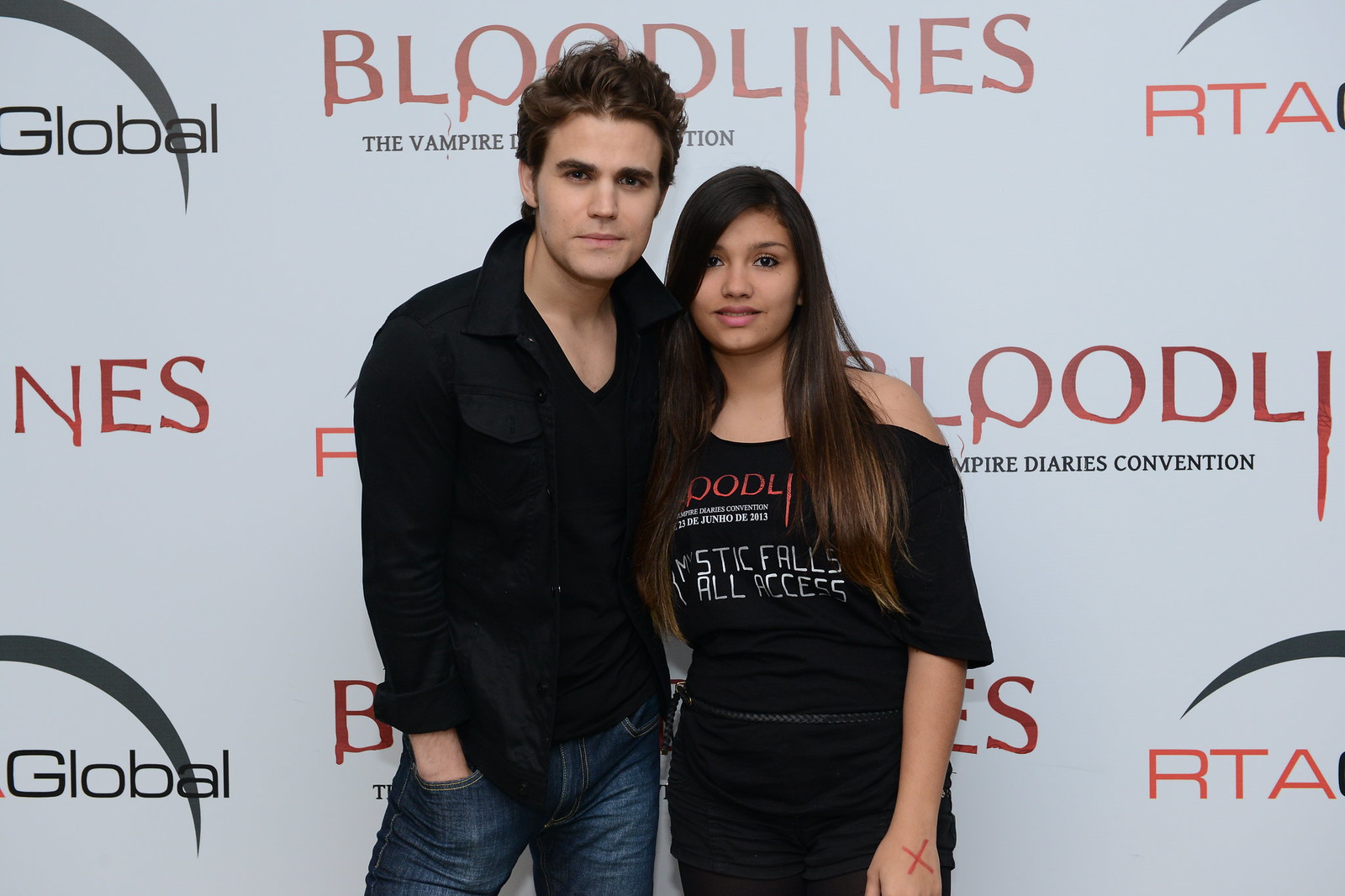In this landscape photograph, a Caucasian man and a Latina woman are posed against a backdrop featuring red and black text that reads "Bloodlines" and "The Vampire Diaries Convention," along with logos for "RTA" and "Global." The man on the left, possibly in his late 20s to early 30s, has wavy brown hair and wears a black, long-sleeved collared shirt, partially rolled up, paired with blue jeans. One of his hands rests casually in his pocket. He appears to be a celebrity, potentially an actor from the "Bloodlines" series. The young woman next to him, likely a teenager or in her early 20s, has long brown hair and a warm smile that reveals a glimpse of her teeth. She is dressed in a black T-shirt with red and white print matching the event's theme and black pants. Her left arm is visible, displaying a red X mark. She seems to be an enthusiastic fan capturing a memorable moment with the actor at this convention-inspired event.